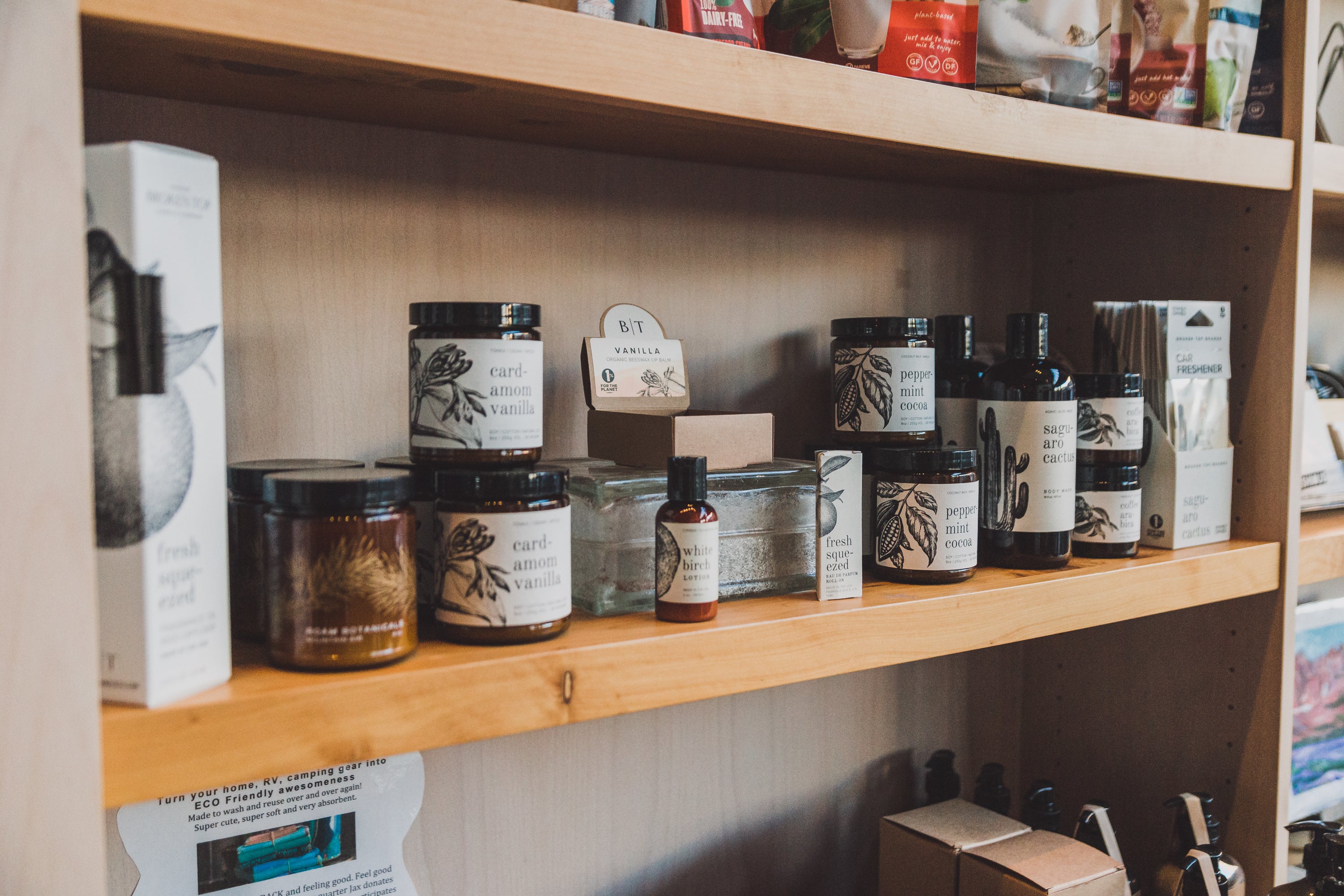This detailed color photograph, taken in a landscape orientation, showcases a collection of herb and seasoning products organized neatly on a set of light beige wooden shelves. The main focus is on the middle shelf, which is slightly wider on the left side due to perspective. This shelf prominently features several dark brown, circular jars with black lids and white labels. The labels on these jars reveal a variety of scents such as "cardamom vanilla" and "peppermint cocoa." Additionally, a smaller brown bottle labeled "white birch" and a rectangular box marked "fresh squeezed" are also visible. Surrounding the main shelf, there are partially visible shelves above and to the right, containing bags and utensils, respectively. The scene captures the meticulous arrangement and diversity of the products, emphasizing their aesthetic appeal and variety.